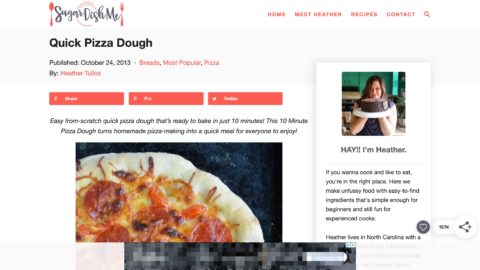This image is a screenshot from a low-quality food blog website, with some blurry fonts making it slightly difficult to read. The overall background, including the top header, is white. On the left side of the header, the logo of the blog is visible. It appears to spell "Sugar Does Me," written in an elegant script that's somewhat hard to decipher. Flanking the logo are a red spoon to the left and a red fork to the right, with a simple, light drawing of a plate situated in the center.

Below the header, a bold black headline announces "Quick Pizza Dough," followed by the publication date, "Published October 24, 2013," indicating the post's age. Under this are three red rectangles, icons for sharing the post on Facebook, Pinterest, and Twitter. The accompanying text describes the recipe: "Easy From Scratch Quick Pizza Dough that's ready to bake in just 10 minutes. The 10-minute pizza dough turns homemade pizza making into a quick meal for everyone to enjoy."

A partial photo of a pizza slice showcasing the dough and pepperoni is embedded within the article. To the right of the text, there is a photo of the blog's author. The photo captions, "Hey, I'm Heather," introduce a white woman with brown hair. She is holding up a chocolate layer cake on a white plate, and from the photo, her elbows and forearms are visible, suggesting a casual, homey kitchen setting with green walls in the background.

Below Heather's photo, a brief descriptor reads: "If you want to cook and like to eat, you're in the right place. Here we make unfussy food with easy to [...] ingredients. It's simple enough for beginners and still fun for experienced cooks," though part of the text is unclear.